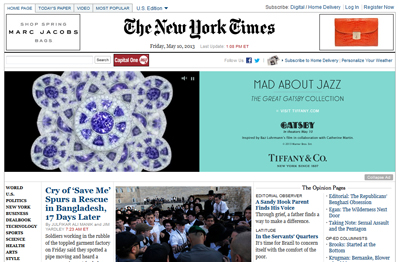The image depicts the New York Times website as it appeared on Friday, May 20, 2013, at 1:08 PM ET. At the top center, the website's header prominently displays the current date and time. On the far right side of the header, there is an advertisement for a red clutch purse. Additionally, an advertisement for Marc Jacobs's Spring collection appears on the far left.

Below these advertisements, occupying a central position on the webpage, is a featured article titled "Man About Jazz: The Great Gatsby Collection." To its immediate left is an image of jeweled gears, presumably part of the same collection. Directly below this central section, another major article is prominently displayed, with the headline "Cry of 'Save Me' Spurs a Rescue in Bangladesh 17 Days Later." Accompanying this article on the right is a photograph showing a group of people, mostly dressed in white shirts, with some officials situated at the front, likely depicting a scene related to the Bangladesh rescue.

To the right of the main articles, there is a section dedicated to opinion pieces, labeled "The Opinion Pages," featuring about five separate articles clustered together. These elements create a comprehensive snapshot of the New York Times' website layout on that particular day.